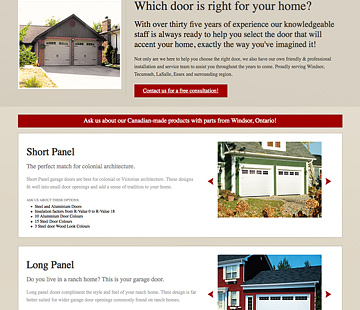This screen capture showcases a series of advertisements focusing on garage doors, presented on a tan background. The top image features a brick house with dual tan garage doors, complemented by a gray roof and lush green foliage. The driveway in front highlights a black banner with the text: "Which door is right for your home? With over 35 years of experience, our knowledgeable staff is always ready to help you select the door that will accent your home exactly the way you imagine it." Below, a paragraph of black text provides additional details, ending with "Contact us for a free consultation" in striking red and white font. A red banner beneath urges viewers to "Ask us about our Canadian-made products with parts from Windsor, Ontario."

The second image displays a green house with two white garage doors, flanked by red arrows on both sides. This image is labeled "Short Panel," accompanied by an explanatory paragraph that highlights its suitability for colonial architecture.

The final image shows a red house with white shutters and a white garage door. Gray shingles cover the roof, and similar red arrows point towards the garage door, labeled "Long Panel." Text below this states: "Do you live in a ranch house? This is your garage door." Despite the small and somewhat hard-to-read font, the overall message emphasizes the range of garage door styles suitable for different architectural designs.